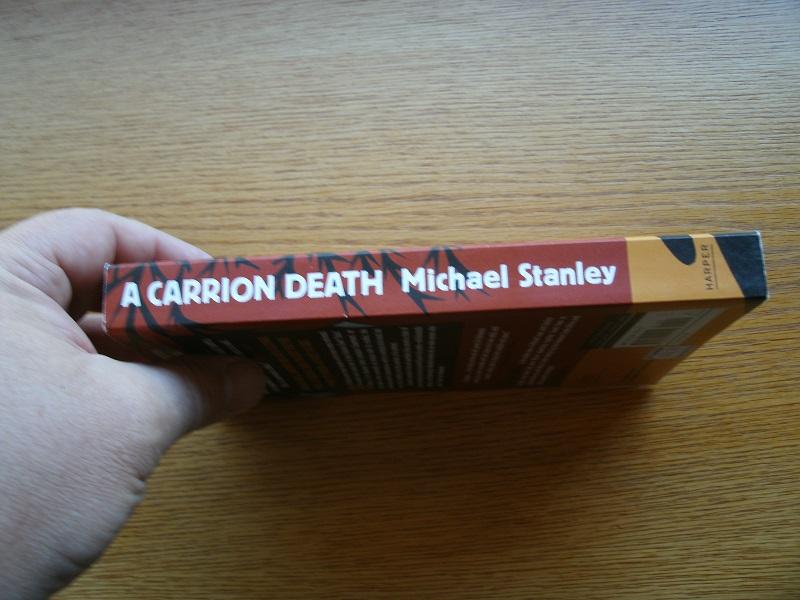The image features a close-up view of a hand, specifically the thumb and first finger, grasping and holding up a paperback book titled "A Carrion Death" by Michael Stanley. The book is positioned sideways, making the title legible along the spine. The cover predominantly displays a red background, adorned with dark branches and leaves. The text on the spine is written in white, with "A Carrion Death" in all capital letters, and "Michael Stanley" below it. At the bottom of the spine, the word "Harper" is also written in white and underlined. The background of the image includes a wooden desk or table with a horizontal grain pattern. The hand holding the book is fair-skinned, and there is a visible shadow below the book, suggesting it is being held inside a home.